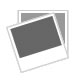This screenshot from a cell phone features a predominantly white background. At the top, starting from the left, black text indicates the time as 2:13. To the far right, there are connectivity bars, a Wi-Fi symbol, and a battery life indicator displayed in sequence. Below this, a series of icons is arranged from left to right: a left-pointing directional arrow, the CJH emblem centered, a small shopping cart icon, and finally, a screen icon with an arrow pointing towards the upper right corner.

Directly beneath these icons, on the left side in black text, the phrase "in the box" is displayed, followed by an image of a DJI RC Pro remote controller. This remote is black, featuring white indicators on the top buttons, and a black rectangular screen. The text "DJI RC Pro x 1" is written below the image. Further down, there is a picture of a USB 3.0 Type-C cable curved in a 'C' shape, with the description "USB 3.0 Type-C cable x 1" beneath it. To the right of this text is an upward-pointing directional arrow.

Towards the bottom of the screenshot is a circular icon showing a person with short black hair, wearing a black shirt. Beneath this icon, the price is stated as "US dollars $1,199." At the very bottom of the screen, a prominent button reads "Add to Cart."